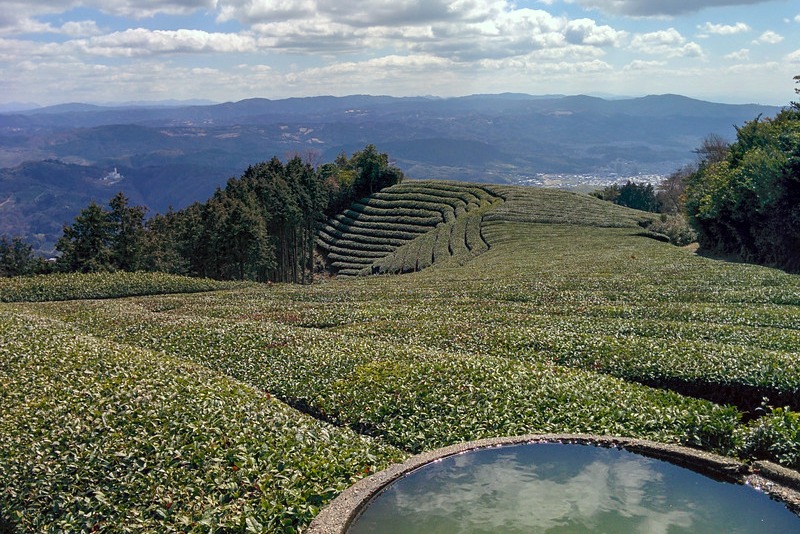High atop a mountain summit, the expansive landscape stretches out before us, revealing a distant horizon dominated by a majestic range of undulating mountains. The sky above is a serene blue, sporadically adorned with fluffy, white clouds casting gentle shadows on the scene below. Directly in front of us lies a unique grassy expanse, characterized by long, neatly arranged columns of grass that resemble contiguous hedgerows, creating a striped pattern cascading down the sloping terrain. Flanking this grassy area are the tops of towering trees, framing the central view. In the very foreground, a charming circular pond with a meticulously crafted stone border adds a touch of tranquility to the captivating panorama.